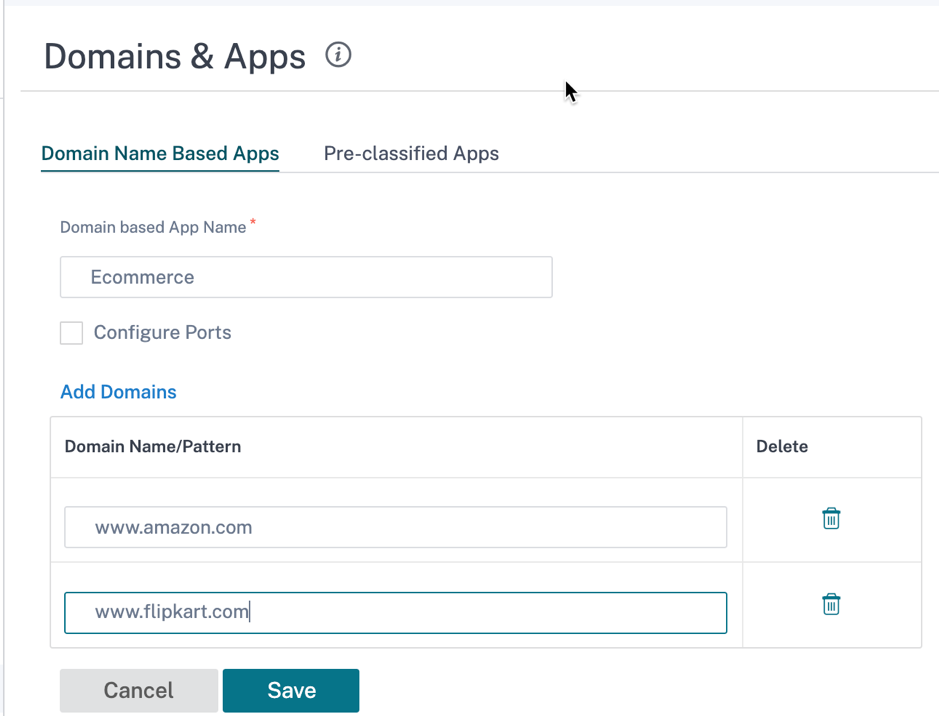In the image, there appears to be a screenshot of a webpage or a computer application interface with a predominantly white background. 

At the top left corner, there is a large, non-bold text in black font that reads "Domains & Apps." Beside this text is an outline of a circle with the letter "i" in the middle. 

Directly below this text, spanning from left to right, is a very thin, gray line. Positioned towards the middle-right section of the interface is a black mouse pointer.

Further below, on the left side, there is a smaller blue text with an underline that reads "Domain Name Based Apps." Adjacent to this text, in an unselected state, it says "Pre-Classified Apps."

Underneath "Domain Name Based Apps," in a lighter gray font, the words "Domain Based App Name" are displayed, accompanied by a red asterisk appearing diagonally off the "E." Within the search box below this heading, the word "e-commerce" is written in a light gray color in a mix of uppercase and lowercase letters.

Below the search box, there is an unchecked box next to the words "Configure Ports."

Further down, in blue text of the same size, it says "Add Domains," followed by a larger box sectioning off different areas. 

Under "Add Domains," there is smaller black text that reads "Domain/Pattern." Towards the far right, there is a vertical line with the word "Delete" written in black to its side.

Beneath this, towards the left side, there is a box containing the text "www.amazon.com" in gray font. To the right of this text, underneath the word "Delete," there is an icon of a blue trash can. Below this, there is another instance of the blue trash can icon.

To the left of this section, there is another search box highlighted with a blue outline, containing the text "www.flipkart.com." Below this box, there are two closely positioned gray buttons: one labeled "Cancel" in black text and the other, smaller box labeled "Save" with the text in white.

This constitutes the detailed layout of the screenshot.